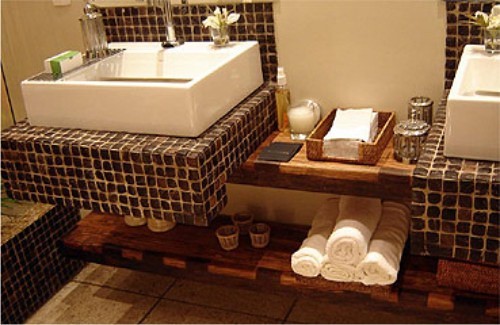The image depicts a horizontally oriented, casually taken photo of a bathroom interior. The bathroom, with the atmosphere of a serene spa, features two white sinks separated by a small ledge. Each sink is adorned with a soap dispenser and a small flower, enhancing the tranquil ambiance. Below the sinks, neatly rolled towels are stacked on top of each other, contributing to the organized and peaceful setting. The backdrop showcases dark brown tiled backsplash, adding a touch of elegance to the scene. Overall, the photo exudes a sense of calm and serenity, reminiscent of a relaxing spa environment.